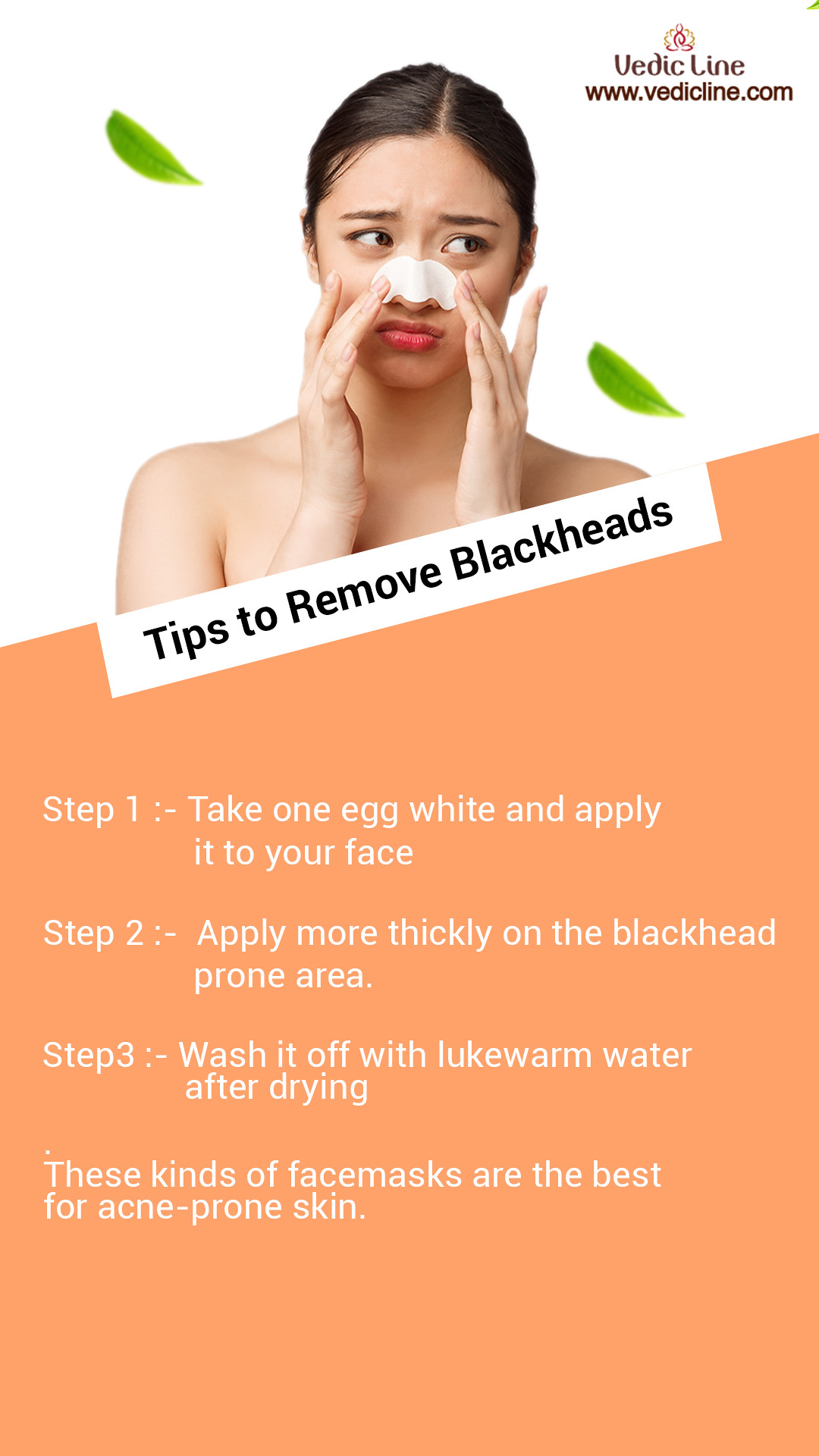This image is an informational poster from Vedicline (www.vedicline.com) featuring beauty tips on removing blackheads. Centered prominently is a computer-generated woman with dark black hair, applying a blackhead nose strip to her face, looking worried and glancing to the right, with green leaves positioned on either side of her. She appears unclothed, visible from her shoulders up. The poster, set against an orange background, reads "Tips to Remove Blackheads" in a white text box. Below, step-by-step instructions in white lettering detail: Step 1: Take one egg white and apply it to your face. Step 2: Apply more thickly on the blackhead prone area. Step 3: Wash it off with lukewarm water after drying. The poster concludes that such masks are ideal for acne-prone skin.